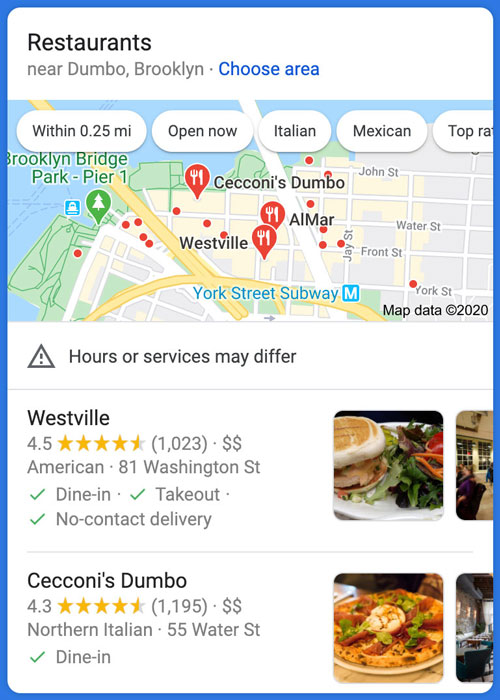The image captures a detailed view of a cell phone screen showing a restaurant search near Dumbo, Brooklyn. At the top, the screen displays the heading "Restaurants" and underneath, it specifies "Near Dumbo, Brooklyn." The phrase "Choose area" is highlighted in blue, indicating it is clickable. A map of Brooklyn dominates the scene, peppered with various pins indicating restaurant locations. These pins, depicted with a fork and knife icon, symbolize eateries. A prominent green pin marks a pier location.

Towards the bottom of the screen, a cautionary triangle with an exclamation point inside signals that "hours or services may differ." This is followed by listings of nearby restaurants. First on the list is "Westville," rated at 4.5 stars with 1,023 reviews. It indicates a moderate pricing with two dollar signs and describes the cuisine as American. The address is noted as 81 Washington Street, offering dine-in, take-out, and no-contact delivery services.

Next is "Ccioni's Dumbo," boasting a 4.3-star rating from 1,195 reviews. It also shows two dollar signs, identifying it as a Northern Italian restaurant located on Water Street, providing dine-in service only. Accompanying the descriptions, several food photographs from both restaurants are displayed, giving a visual taste of what they offer.